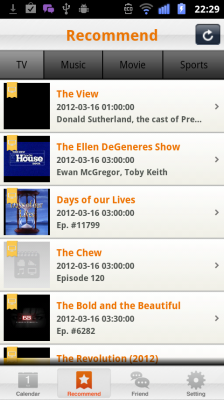The image is a low-quality screenshot of an app running on an old Android phone. The device's dated interface is evident, with blurred pixels and low resolution. At the top of the screen, status icons include the Android logo, Wi-Fi signal, cellular signal bars, and a charging indicator. The time displayed is 22:28. Below the status bar, "recommend" is prominently shown in orange text, accompanied by a reload page icon to the right.

The main section is divided into categories labeled TV, music, movie, and sports, each with a gray rectangular background. The TV category is currently selected, displaying a list of shows including "The View," "The Ellen DeGeneres Show," "Days of Our Lives," "The Chew," "The Bold and the Beautiful," and "The Revolution 2012." Show titles are in orange font, with additional details such as duration, episode numbers, and cast names in gray font beneath them. Each show title is flanked by an arrow on the right side and a relevant logo on the left.

At the bottom of the screen, there are additional navigation tabs labeled calendar, recommend, friend, and setting.